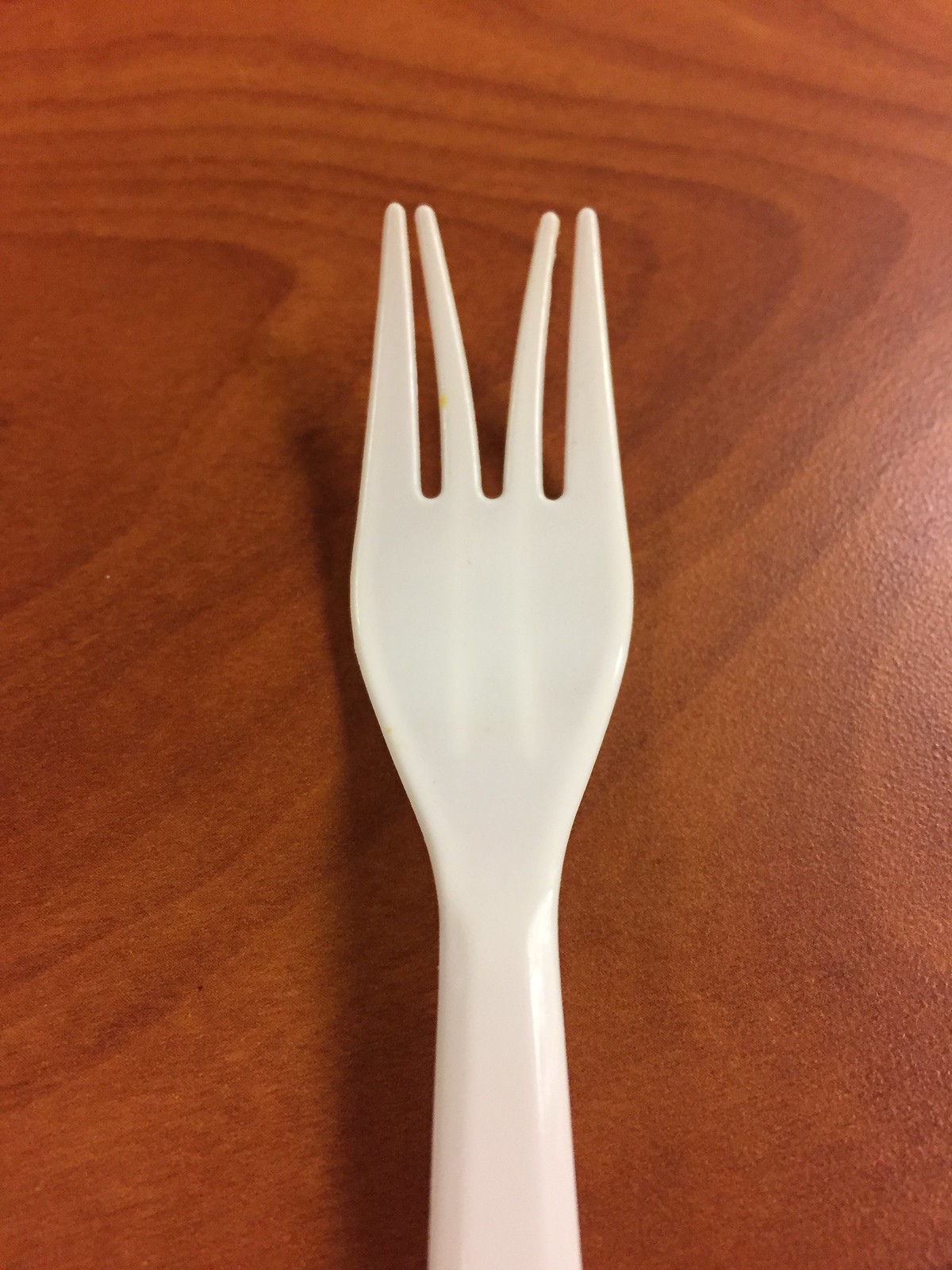This detailed image captures a close-up view of a white plastic fork placed on a brown wood grain table, though it’s unclear if the table is real wood or Formica. The fork is positioned vertically and centered in the frame, with a light source illuminating the right side, casting a distinct shadow beneath. The fork features four tines, with the two middle tines notably bent outward, creating a noticeable gap between them. The photograph is taken from above, emphasizing the intricate details of the plastic material, which one might overlook in everyday use. Despite the detailed close-up and lighting, there is no context indicating whether the image was taken in a restaurant, home, or workplace.